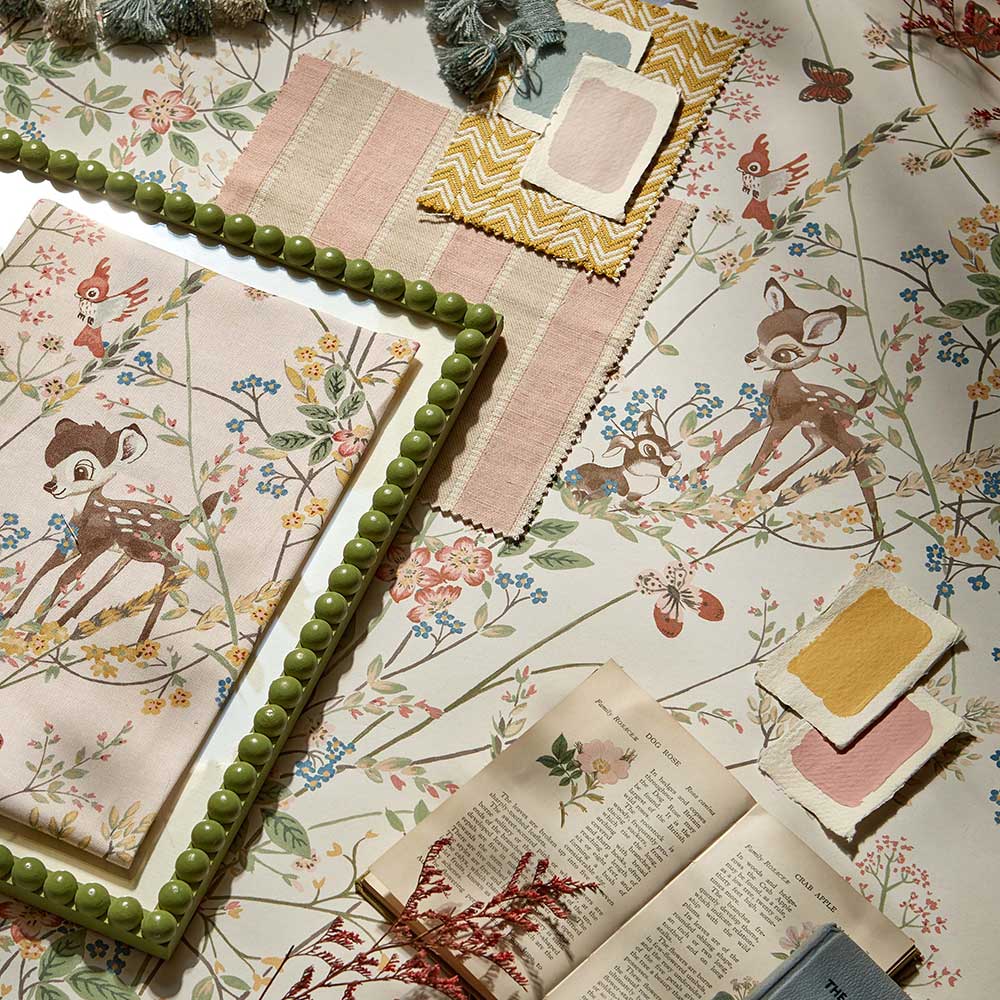A photograph captures a charming scene from a little girl's room, showcasing an assortment of items laid out on a printed tablecloth featuring a repeated scene from the movie "Bambi." The tablecloth, predominantly white, is adorned with images of Bambi, Thumper, and a variety of birds and butterflies amidst a backdrop of flowers, rendered in soothing browns, blues, and rose colors. Several fabric swatches lie on the tablecloth, hinting at a room renovation project. These swatches include patterns of purple, pink, striped pink and beige, and a golden-white chevron design. 

At the center, an olive green beaded frame holds a fabric piece of the same Bambi print, though it appears not to be permanently mounted. To the lower right, an open book about flowers displays a pinkish-red dried floral piece on its pages, while a pink flower with green leaves decorates the upper left of the book. Surrounding these items are various decorative elements in gold and pink, adding a touch of whimsy and sophistication to the scene. A light pink and beige cloth rests towards the top of the photograph, completing this delightful and detailed tableau.